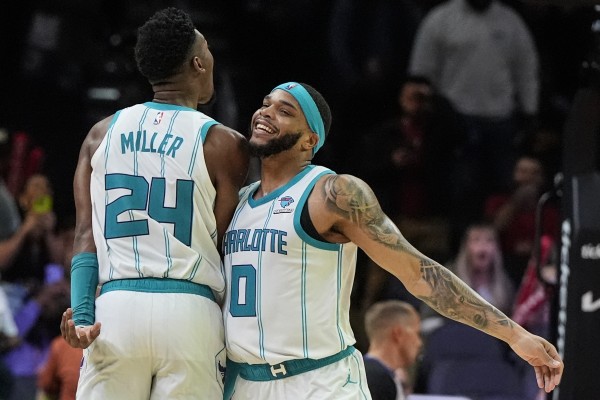The photograph captures an exuberant moment between two Charlotte Hornets basketball players, identifiable by their white jerseys with light blue accents and the name "Charlotte" displayed prominently. The player on the left is Brandon Miller, wearing jersey number 24, with "Miller" and the NBA logo visible on his back. Miller sports a team-colored wrist strap and stands with his left arm raised, possibly in celebration. The player on the right, number 0, is Miles Bridges. He faces the camera with a radiant smile, wearing a matching headband and displaying a sleeve of gray tattoos on his left arm, which he extends outward. Bridges, with his chin slightly resting near Miller's right arm, showcases a well-groomed beard. Both athletes appear overjoyed, hinting at a positive moment in the game. The background features a blurry crowd, adding depth to the image, with one discernible man in a white shirt.